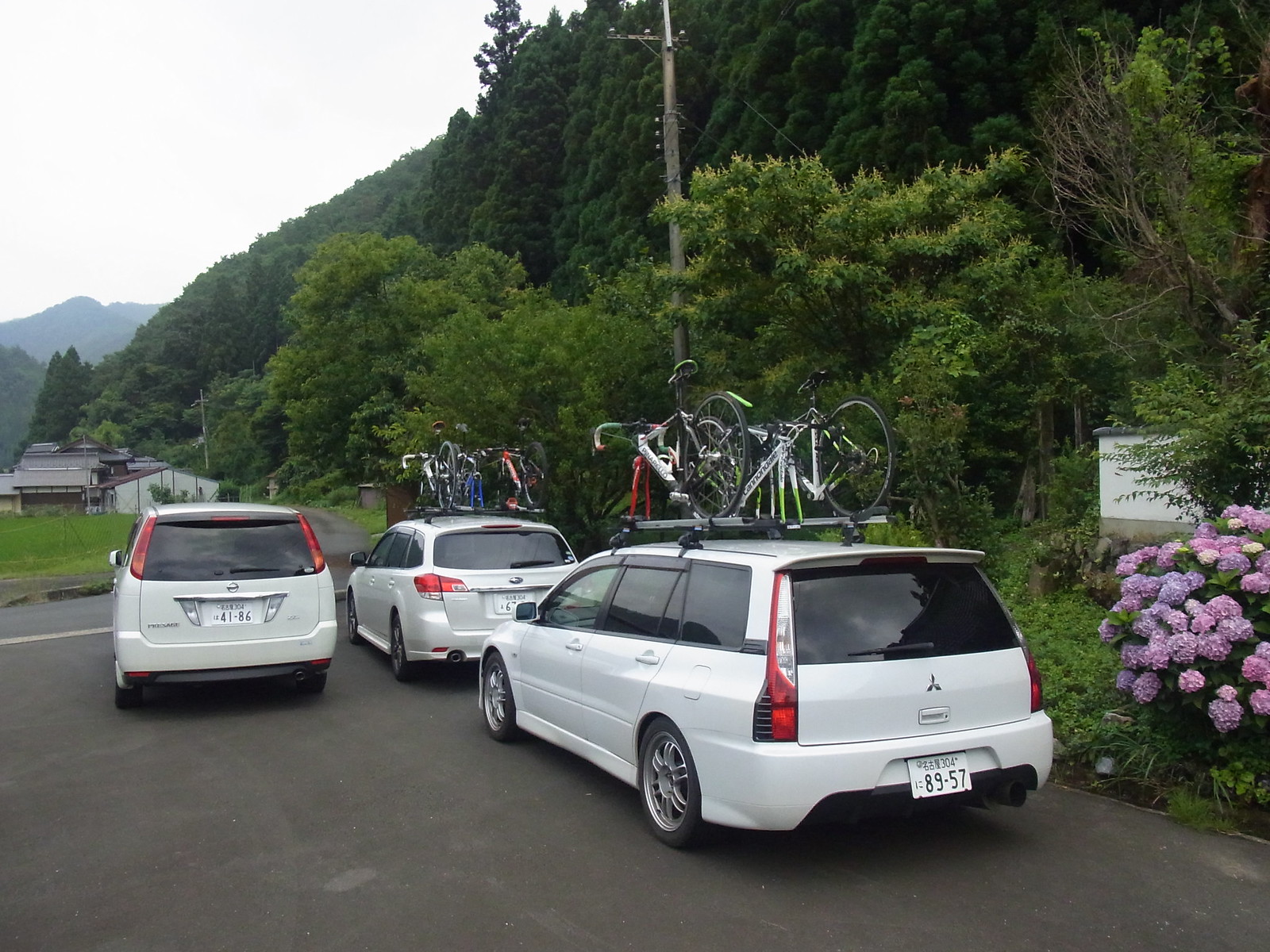In this photo, we observe three white station wagons or vans parked in an asphalt parking lot, likely situated in a park. The cars appear to be different models: one is identified as a Mitsubishi, another as a Subaru, and the third as a Nissan. Each vehicle features white license plates with low, four-digit numbers that may not be real. The two cars on the right are parked next to each other and boast bicycle racks on their roofs, each carrying three bicycles. The third car is positioned behind the rightmost forward vehicle.

The parking lot is bordered by dense woods on the right, creating a wall of greenery. In the background, we can see an electrical pole near the edge of the forest and another farther down by a building. A dirt road leads from the front of the parked cars to a complex-looking single-story structure. Far beyond the immediate scene, a rounded hill or small mountain is visible, completing the natural scenic backdrop.